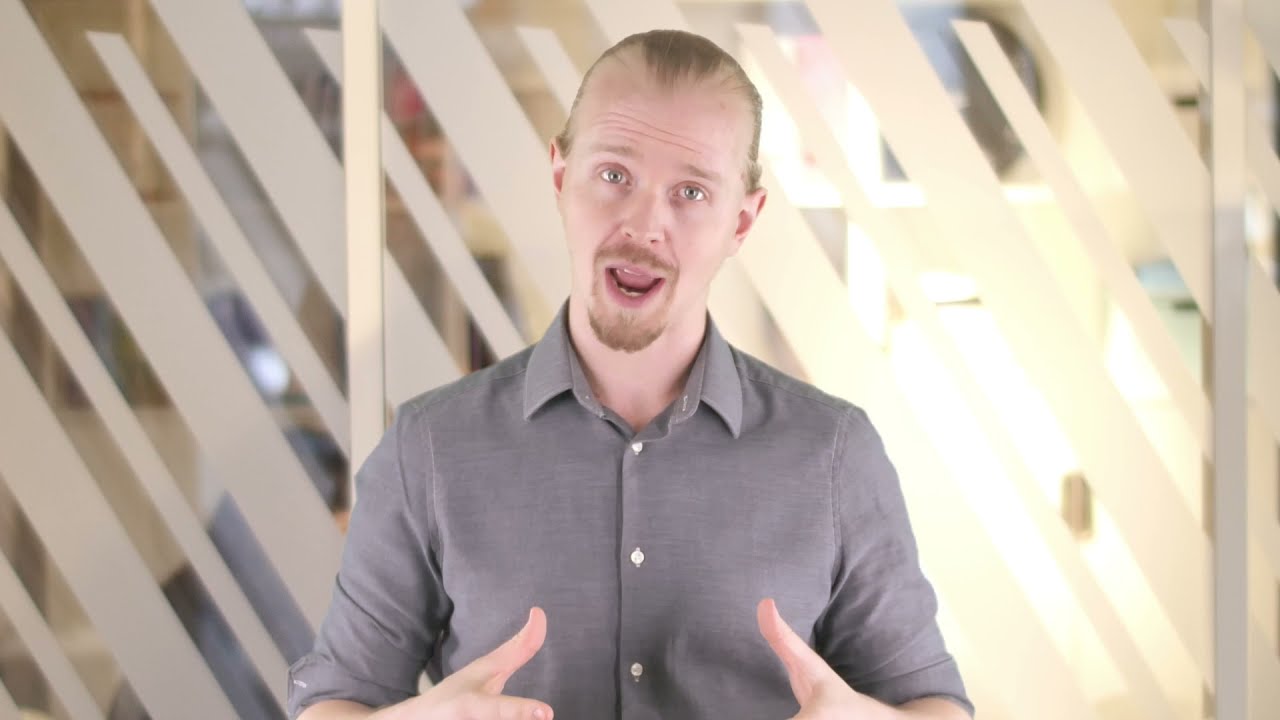The photograph captures a pale-complexioned white man with a receding widow's peak hairline, light blue eyes, and long, blonde hair tied in a ponytail. He has a blonde goatee and mustache. The man is centrally positioned, making direct eye contact with the viewer. He is wearing a gray button-up shirt with white buttons, and the sleeves are rolled up to his elbows, revealing his forearms and fingers. His mouth is open as though he is speaking, and his hands are raised in front of him, suggesting he is in the middle of gesturing. The background consists of a glass wall with cream or light beige diagonal stripes from the top left to the bottom right, implying indoor office settings. This glass panel offers a faint view of indistinct blue and beige shapes, possibly indicating other parts of the building.